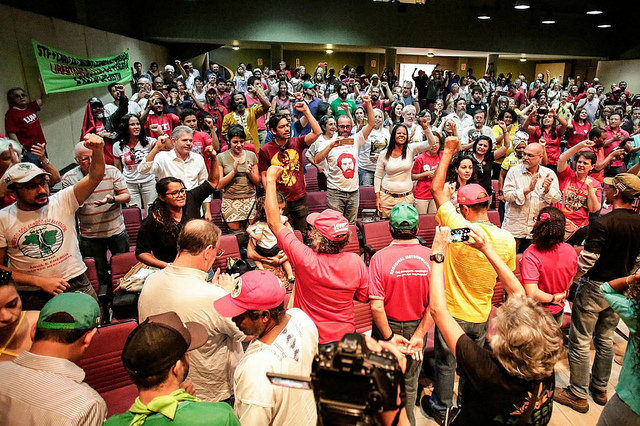In this photograph, a large room filled with people is depicted, suggesting a dynamic and possibly festive or rally-like atmosphere. The room features a dark-colored ceiling with pot lights and various red padded folding chairs, though nearly everyone is standing. The crowd, which appears to number in the hundreds, is seen cheering with joy, unified by the simultaneous raising of their right fists. This diverse assembly includes men and women of various ethnic backgrounds, many casually dressed in multicolored clothing and baseball caps, predominantly in red or green. Several participants are donning a distinct pinkish-red T-shirt, hinting at a shared cause or event. Along the far left wall, two individuals hold up a green banner with writing, adding to the sense of purpose in the gathering. In the front, numerous people, likely photographers, are capturing the moment with a variety of cameras and cell phones, facing the crowd. Red padded folding chairs are visible, though they are unoccupied as the crowd stands in celebration. An older digital camera on a stand suggests the photograph might capture a historical moment, adding to the sense of significance that permeates the scene.